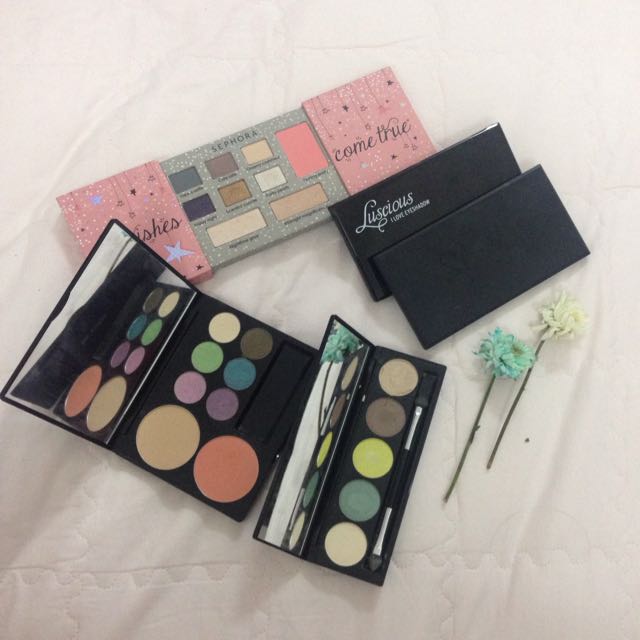The vertical rectangular image depicts a detailed display of various Sephora makeup products arranged on a gray background, possibly a granite or marble countertop with darker gray streaks. Central to the image is a large pink rectangular package from Sephora with the phrase "wishes come true" inscribed on it, showcasing a selection of makeup items including blush and eyeliner. To its right, there are two black makeup compacts featuring mirrors inside their lids. On the far right of the image, two applicators lie ready for use. Scattered among the makeup are two sleek black compacts, one of which has "Luscious" written in silver script. Additionally, there are floral accents: two flowers on thin green stems—one light blue and one white—adding a delicate touch to the display. In total, two open makeup boxes reveal a variety of colorful eyeshadows arranged in circles, complemented by mirrors and brushes, reflecting the brand's attention to detail and aesthetic appeal.